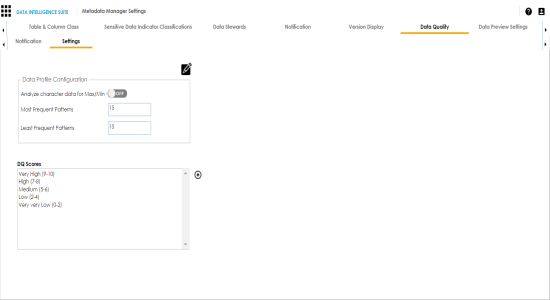The image displays a blurred printout that appears to be dominated by data, making it largely undecipherable. At the top of the page, there are seven clickable options, with the one on the far right side highlighted in gold. Additionally, another choice on the left side is also highlighted in gold. Although the contents can't be fully explained due to the blur, it is evident that the printout includes numerical data potentially representing scores categorized as very high, high, medium, low, and very low. The document includes references to "data-specific conjugation" and comprises various tables and color-coded elements. Some portions of the text might be in languages other than English.